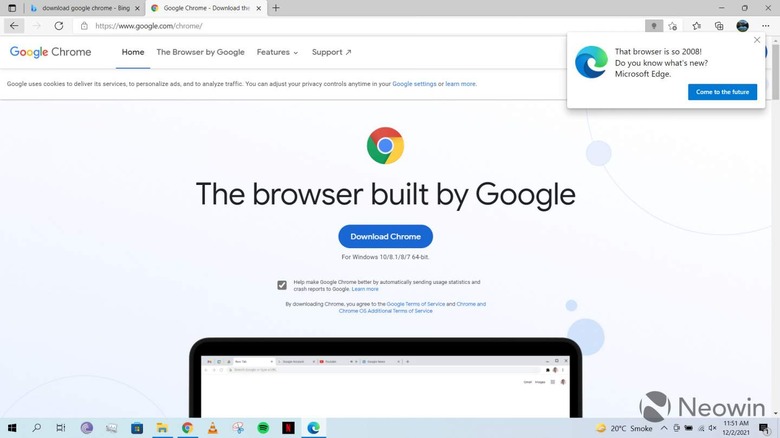This is a screenshot of the Google Chrome browser. At the top of the screen, there are two visible tabs. The URL bar below indicates that the user is on google.com/chrome. The main content displays the Google Chrome homepage.

In the top left corner, the page header reads "Google Chrome," accompanied by Google's colorful logo, which features the colors green, red, yellow, and blue. The top menu bar contains black links labeled "Home," "The Browser by Google," "Features," and "Support."

Additionally, there is a pop-up window in the top right corner displaying the Microsoft Edge logo. The text in the pop-up reads, "That browser is so 2008. Do you know what's new? Microsoft Edge. Come to the future." Beside this message, there is a blue button.